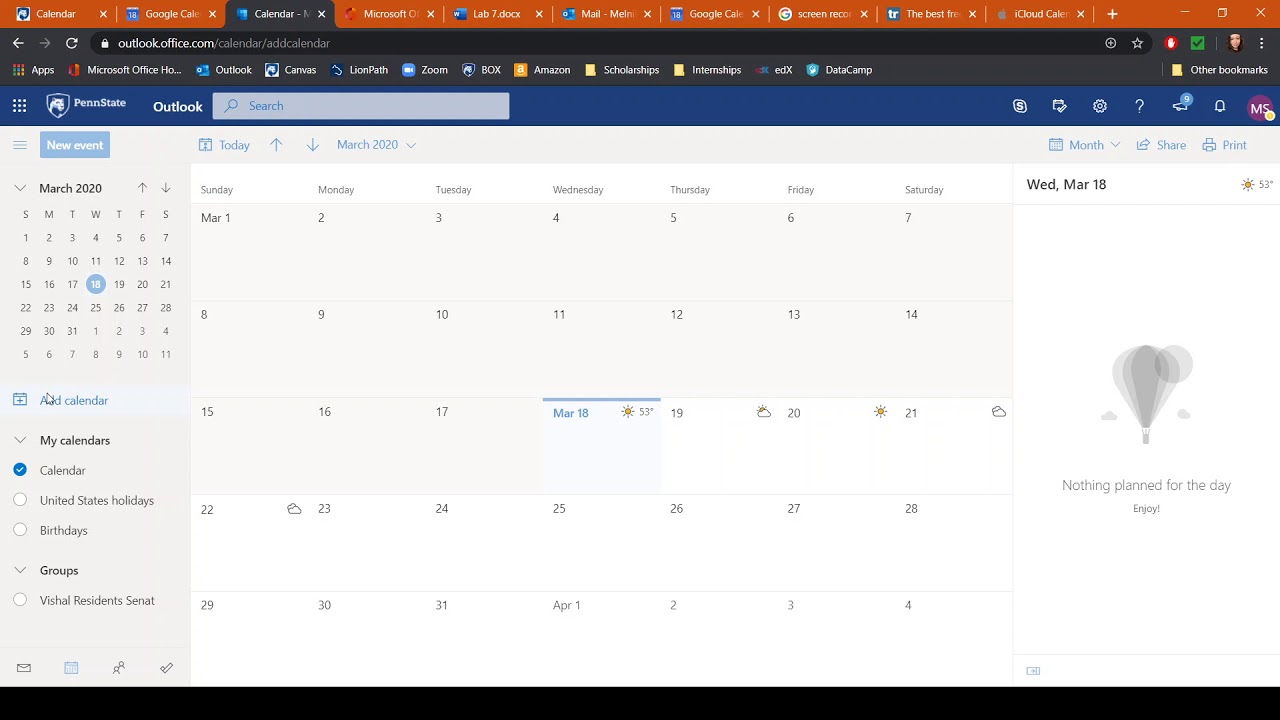The image displays a computer screen showcasing a calendar interface on Outlook Office. The top bar is mainly orange, except for the selected 'Calendar' tab, indicating the active view. Starting from the left, the navigation tabs are laid out in the following order: Calendar, Google, Calendar, Microsoft, followed by six additional tabs.

Below this is a gray address bar showing the URL 'outlook.office.com'. Underneath, a menu is present, followed by a prominent blue line that spans the width of the screen, featuring an Outlook logo and a search bar.

The main section of the screen displays a white background calendar layout. The layout is divided into a grid with seven columns and five rows, representing the days of the month. The calendar begins with March 1st and extends to April 4th. Each day is neatly boxed, aiding in easy date identification and organization.